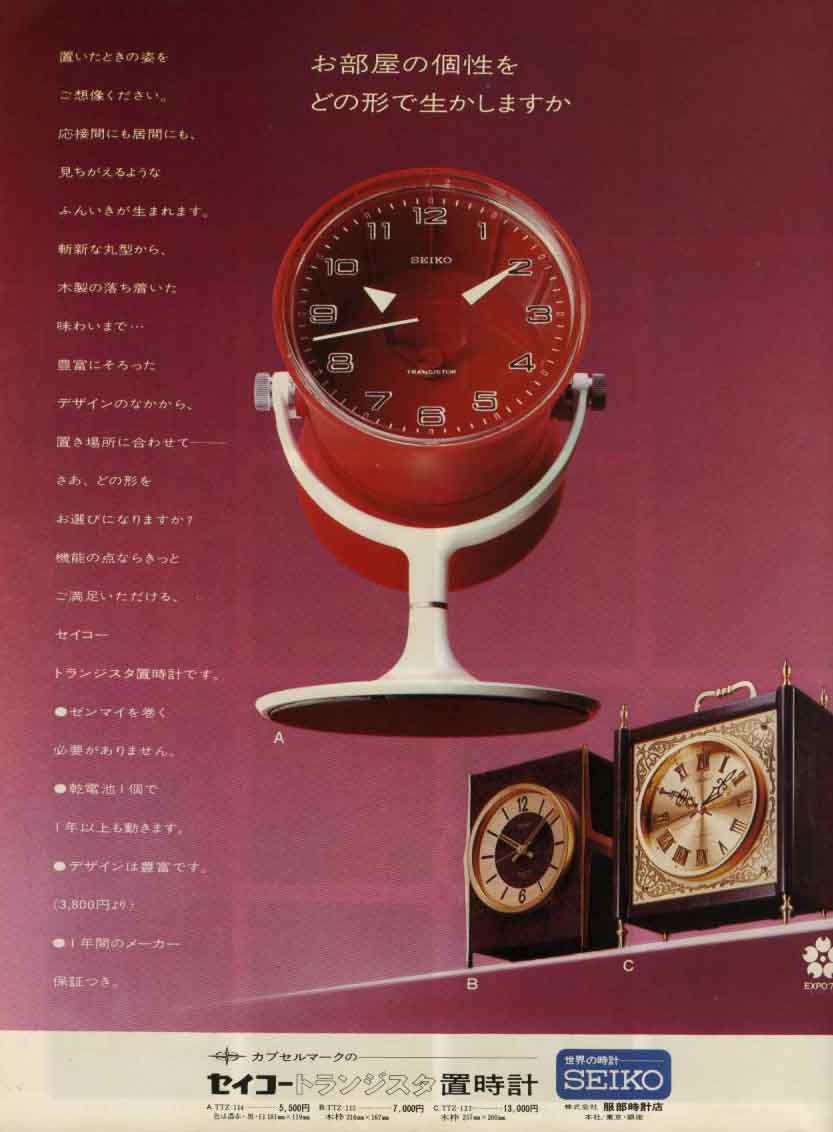The image appears to be an advertisement for Seiko clocks, possibly from an older Japanese magazine. The background is a rich maroon color, with a gradient fading to white towards the bottom left corner. At the center of the image is a striking red desk clock, designed to sit on a white swivel stand. The clock features prominent white hands and a mirrored face. 

Above the clock, two lines of Japanese text, written in a creamy gold color, add an element of elegance to the ad. To the left of the clock, running vertically, is a column of additional Japanese text, also in creamy gold font but smaller in size. 

At the bottom of the image are two Seiko mantel clocks. These clocks have a more traditional aesthetic: one is made of wood with a brown, square body and gold accents around the clock face, while the other has a similar design but appears to be made of laminate. 

Beneath these mantel clocks, a tan strip and a blue box inlaid with the word "Seiko" mark the bottom of the advertisement. The overall effect is a blend of modern and classic styles, showcasing Seiko's range of timepieces against an elegant maroon backdrop.